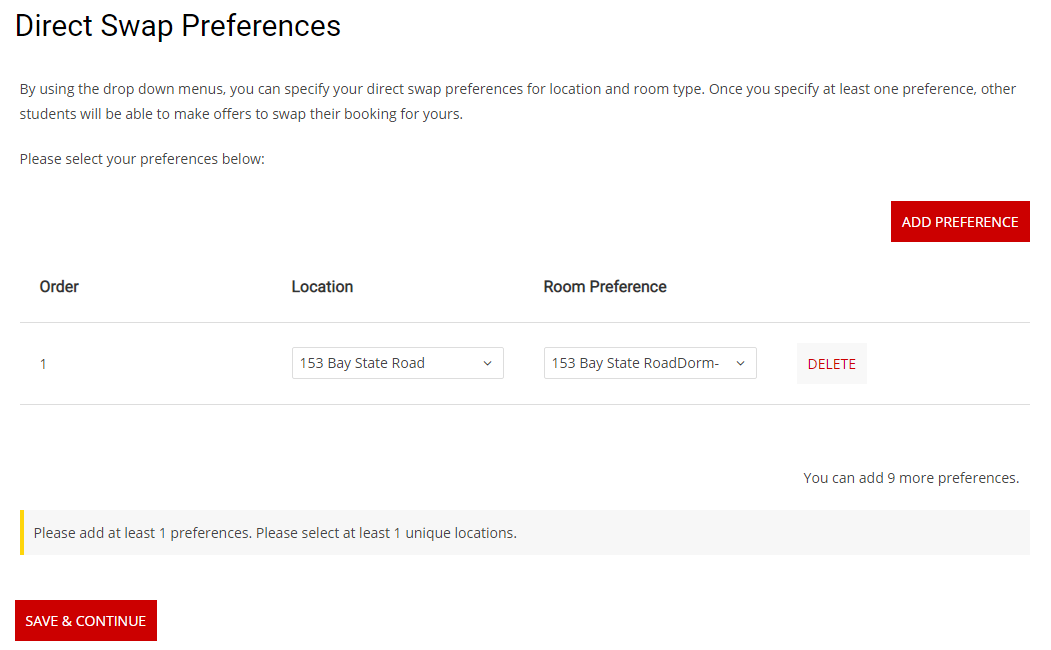Caption: 

The image depicts a webpage or application interface titled "Direct Swap Preferences," prominently displayed in large text at the top left. Below the title, there is a paragraph of standard-sized text explaining the feature: users can specify their location and room type preferences for direct swaps using drop-down menus. By setting at least one preference, students open the opportunity for others to make swap offers on their bookings. 

Under this informational text, a prompt to "please select your preference below" is displayed. On the right side, there is a bright red button labeled "Add Preference" in white text. Below this button, there is a table with columns named "Order," "Location," and "Room Preference," all highlighted in bold black text. 

Within the table, under the "Order" column reads "1," under "Location" it states "153 Bay State Road," and under "Room Preference," it specifies "153 Bay State Road Dorm." Adjacent to these details is a white button with red text labeled "Delete," allowing users to remove this entry. 

Further down on the right, there is an indication that users can add up to nine more preferences. An advisory note at the bottom prompts users to "add at least one preference" and "select at least one unique location." Finally, a red button with white text at the very bottom says "Save and Continue," allowing users to proceed after making their selections.